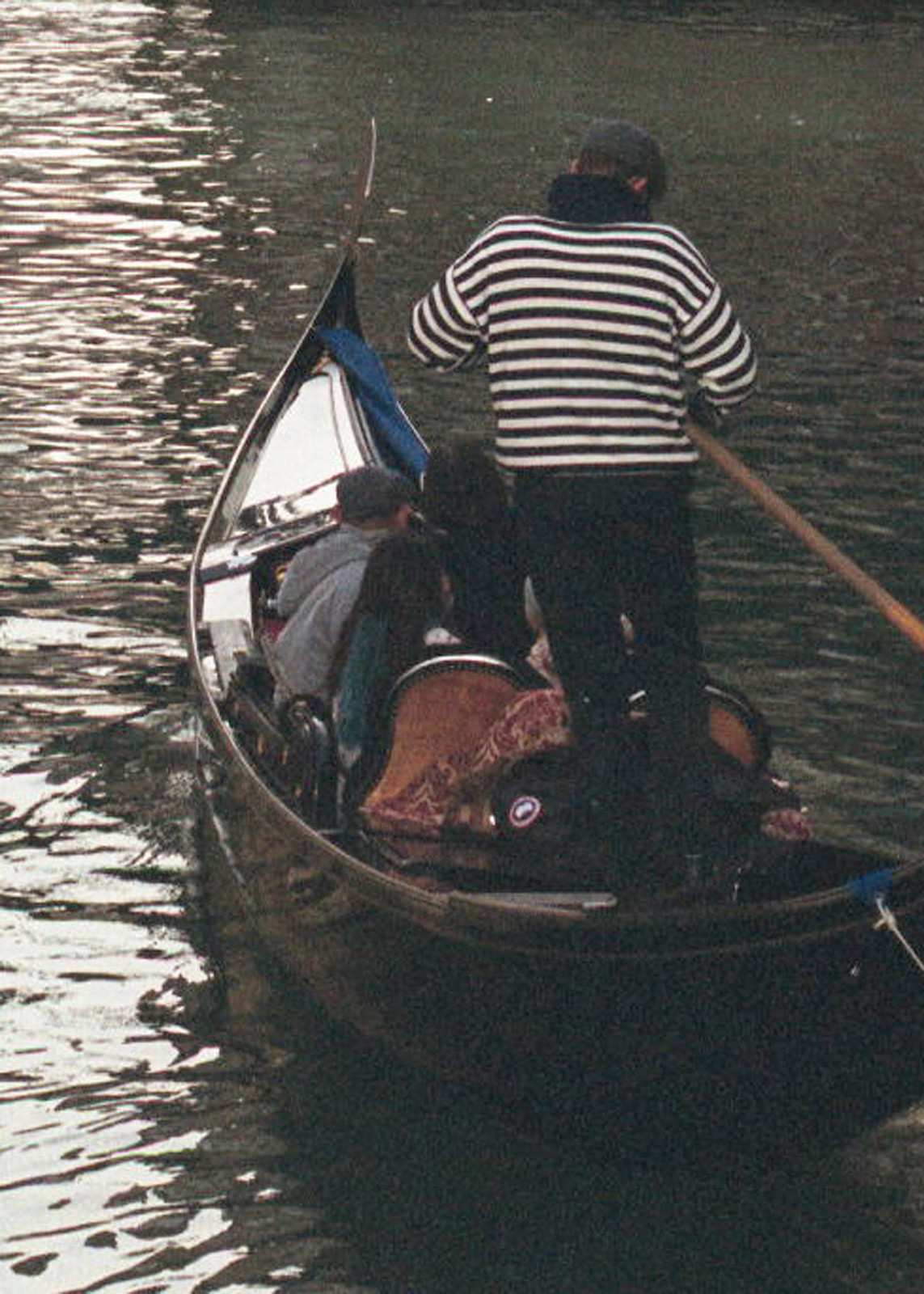This photograph captures a picturesque moment on a gondola ride through what appears to be the canals of Venice. The gondola, which has a sleek, brownish hue with a long-pointed metallic bow, is helmed by a gondolier standing at the rear. The gondolier dons a quintessential black and white striped sweater, black pants, a black scarf around his neck, and a stylish French beret. He holds a long wooden oar, poised to propel the boat through the water which shimmers under the sun, creating a dappled effect on the right side.

In the front part of the gondola, a group of four to six tourists can be seen seated. Despite the chilly atmosphere suggested by their coats, they are likely captivated by the serene and romantic surroundings. Among the tourists, there appear to be two men and two women, all with brown hair, and one of the men is sporting a hat. The image, although slightly dark and grainy, showcases the gondolier momentarily paused, possibly checking his watch, amidst what is presumably a leisurely tour of this iconic locale. In the shadowy background behind the tourists, there seems to be a structure resembling a canopy, adding to the rustic charm of the scene.